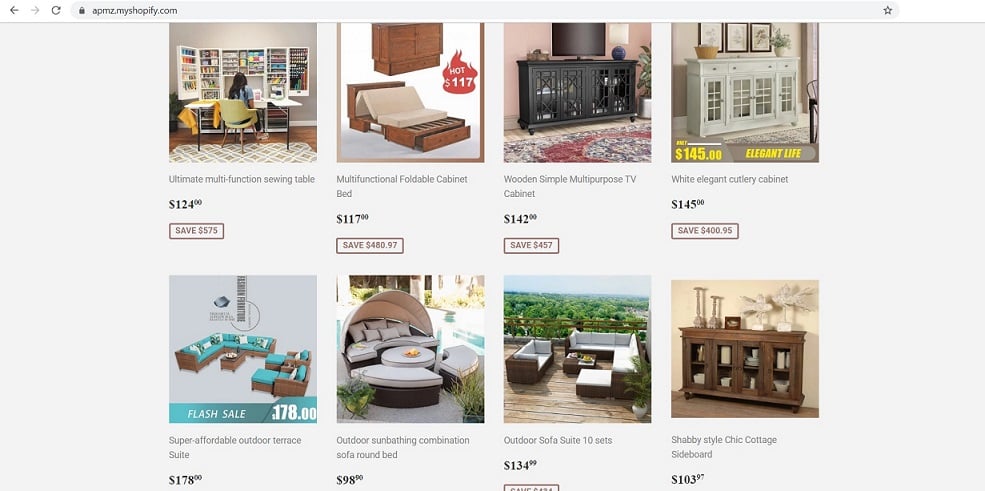Screenshot of a MyShopify.com Shopping Website Displaying Furniture Items

The screenshot captures a MyShopify.com shopping webpage featuring a collection of eight distinct furniture items. The webpage interface is clean and organized, with each item displayed in a grid format. The product assortment includes:

1. A modern wooden desk.
2. A plush, upholstered bed.
3. Two elegant cutlery cabinets.
4. A set of chic outdoor patio furniture.
5. Two additional stylish patio furniture sets.
6. A sleek, contemporary sideboard cabinet.

Beneath each item's image, there is a title succinctly describing the furniture piece. Adjacent to the title, prominently displayed, is the price for the item. Under each price, a savings tag is visible, detailing the discount amount customers can avail of by purchasing through MyShopify.com. The tags make it clear how much buyers can save, adding an appealing incentive for potential customers.